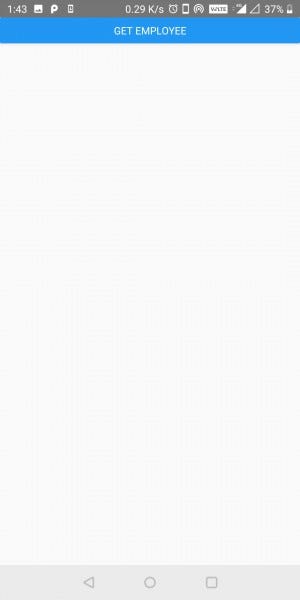The image depicts a screenshot of a smartphone display, showcasing various elements typical of a mobile interface. At the very top, a narrow gray horizontal strip provides essential information, such as active apps, the current time, Wi-Fi connectivity, network signal strength, battery percentage, and possibly indicators for other active features like a timer.

Beneath this, a slightly larger bright blue horizontal rectangle spans the upper quadrant of the image. Centered within this blue strip are the words "GET EMPLOYEE," written in a lighter blue and capitalized, indicating a command or title related to an employee management application or website.

The central portion of the image is dominated by a blank, light gray space, devoid of any text or graphical elements. This empty area extends down to the bottom quadrant, which features a thin, darker gray strip. Superimposed on this strip are three navigation icons commonly found on smartphones: a 'Go Back' button, a 'Minimize' button, and a 'Select' button, which help users navigate the device.

Overall, the screenshot captures a minimalist layout, possibly of a mobile website or application, with a focus on the "GET EMPLOYEE" feature at the top.